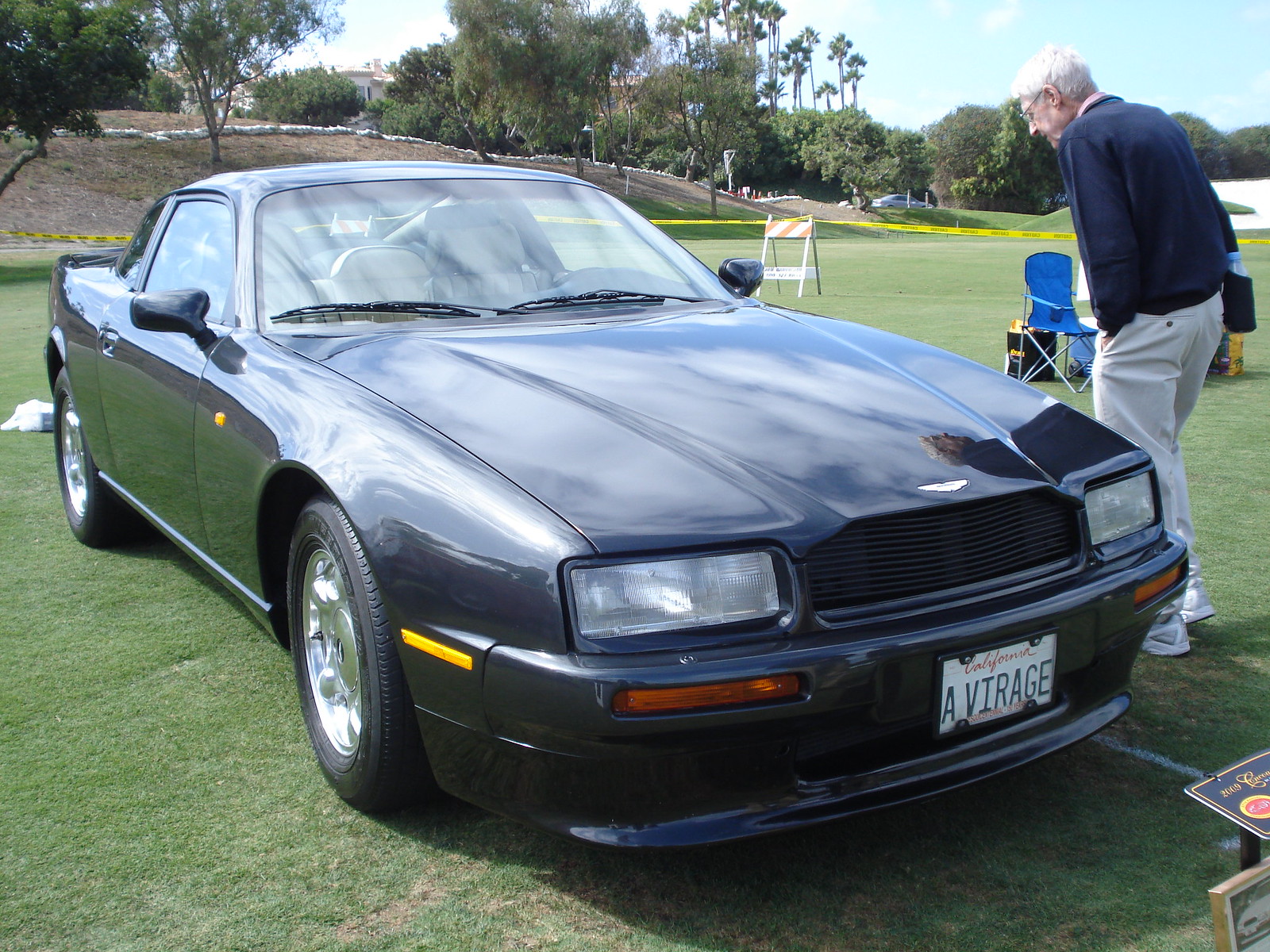In the image, there is a sleek, black Aston Martin coupe parked on a meticulously maintained golf course, its short green grass highlighting the car’s dark, glossy finish. The scene is framed with lush green trees and a large distant building that resembles a mansion, epitomizing a suburban backdrop. The photograph also includes a hill and a sand trap in the background, common features of a golf course. The car, surrounded by a wide boundary of yellow caution tape, is clearly the focal point and features a California license plate that reads "A B I R A G E." 

To the right of the car, but appearing on the left side of the image, an elderly man with gray hair stands hunched over. He is dressed in a navy blue sweater, khaki pants, and white shoes, closely observing the car. A small placard in front of the vehicle suggests it may be part of a car event or display. The overall composition of the image captures the contrast between the refined elegance of the car and the expansive natural beauty of the golf course.